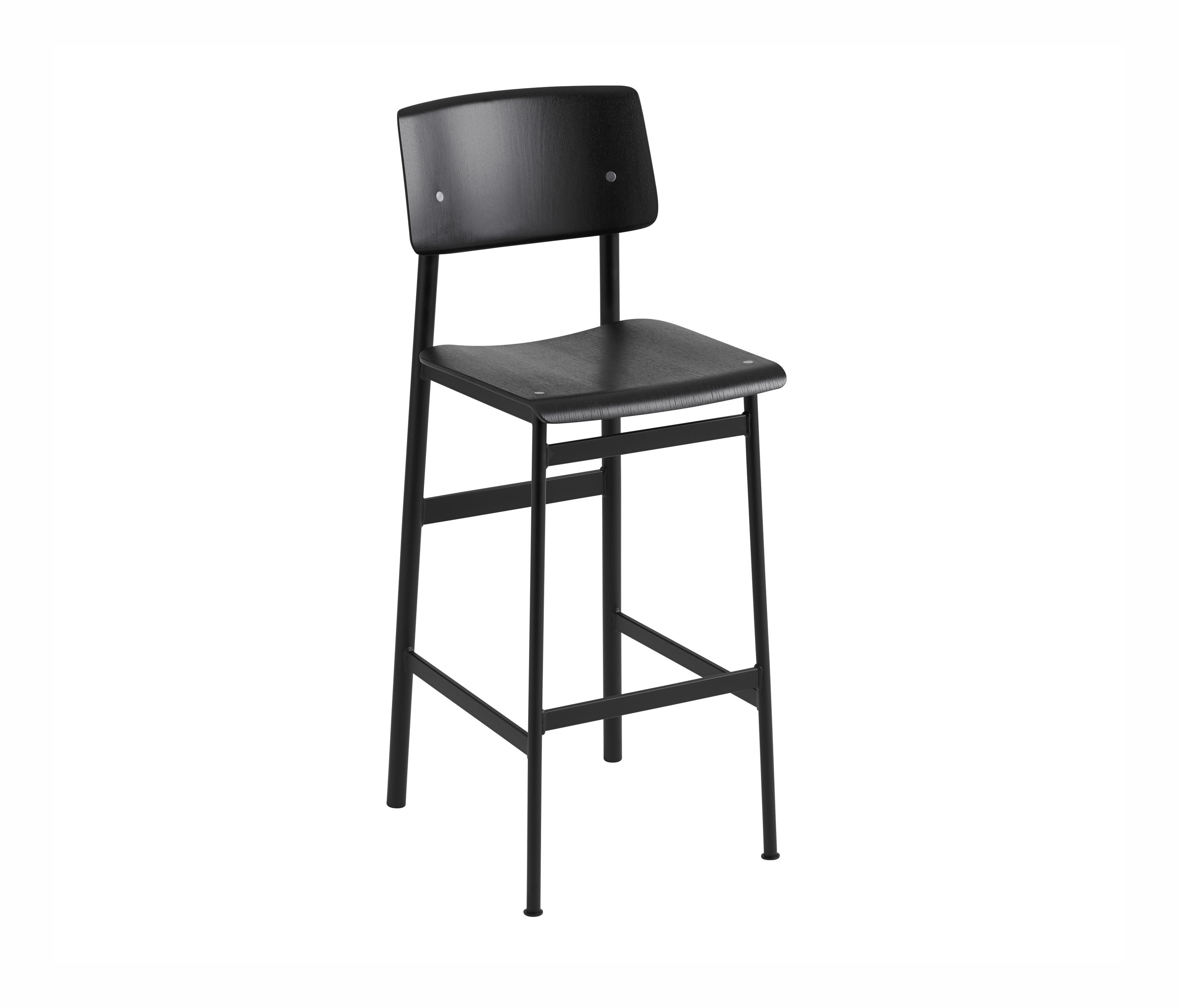The image displays a pixel art depiction of a high bar stool set against a featureless white background that blends seamlessly with the hit page, creating no visible borders. The stool itself is characterized by its contemporary, simple design and consists entirely of black elements, including its long narrow legs, flat seat, and backrest. These components appear to be made from either plastic or wood, painted black. The stool features four iron rod legs reinforced with horizontal braces; three braces connect the legs at the bottom, while two braces are positioned at the top in front, and one at the back. Silver screw heads or rivets are visible at the corners of the seat and attach the backrest to the supports. The stool's minimalistic and clean aesthetic suggests it would be suitable for a high top table at a restaurant, a home bar, or even in a doctor's office where a higher chair might be desired. The stool is angled slightly to the right, giving a clear view of its structural details.